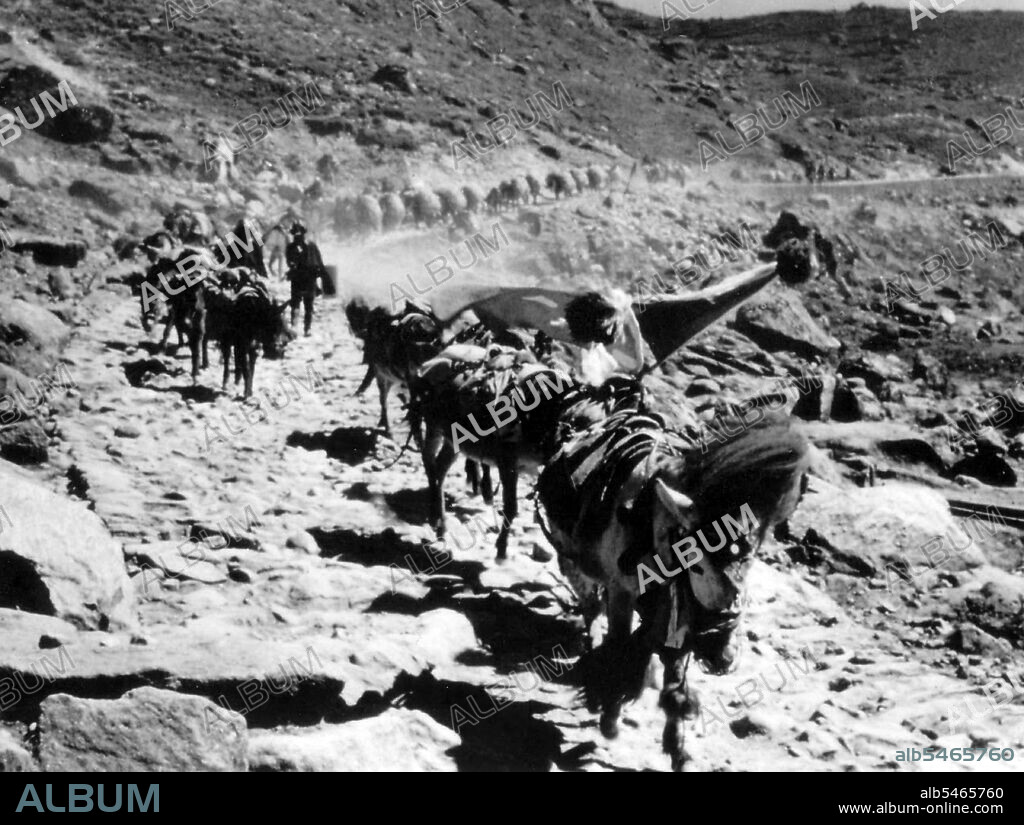This black and white photograph captures a bustling scene of a large caravan traversing a rocky, mountainous trail. The image depicts a long row of donkeys, heavily laden with various goods, making their way carefully along a treacherous path. The mountain, depicted on the left side of the image, contrasts sharply with a sheer drop on the right, adding a sense of danger to the journey. Several people accompany the animals on foot, while a person riding what appears to be a horse can be seen in the background. The trail winds like a 'C' through the landscape, and the overall scene appears historical, likely from the early 1900s, suggested by the attire of the people and the appearance of the animals. The word "album" is lightly watermarked numerous times across the image, and a black strip at the bottom left reads "album," with the bottom right corner displaying "ALB 5465760 www.album-online.com."